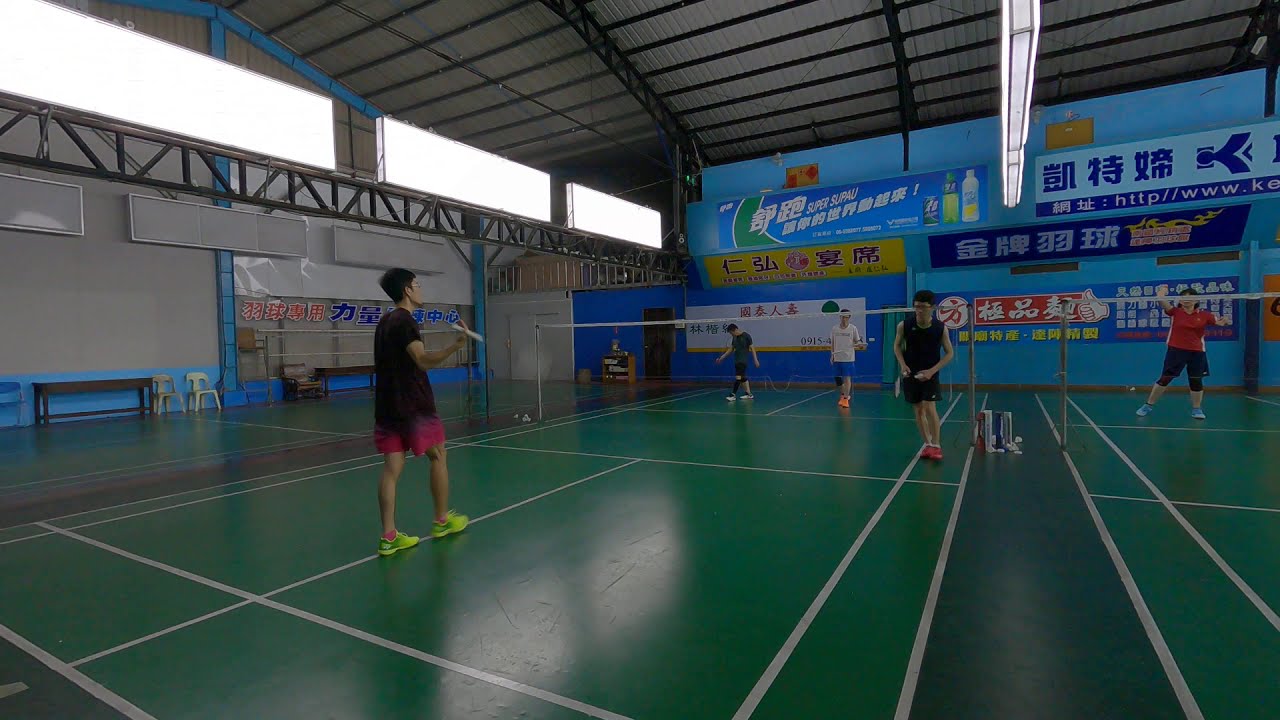The image captures an indoor badminton court with a green surface marked by white lines. There are three courts visible, each separated by nets held up by grey metallic pillars. The ceiling is a complex structure of white metal with black support beams and features rectangular white lights attached to metal support beams. The setting appears to be in an Asian country, inferred from the numerous billboards around the court featuring Asian characters, with one prominently advertising a drink, possibly the local equivalent of Gatorade or Powerade.

In total, there are five players visible. On the left side of the image, one player wears a purple and black outfit with yellow shoes, next to another in a blue shirt and black shorts. Further to their right is a player in a white shirt, blue shorts, and orange shoes. The fourth player on that side wears a sleeveless black tank top with black shorts and red shoes. On the opposite side of the net, there's a lone player in a red shirt. Additionally, there is a woman partially visible at the far right, suggesting more players out of frame. The walls of the building are largely blue, complementing the blue accents in the advertisements.